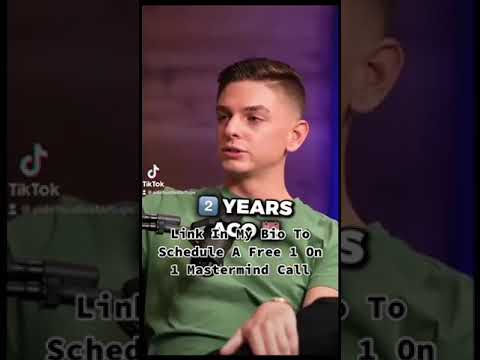The image showcases a young man, possibly in his late teens or early 20s, with short brown hair styled with a buzz cut on the side. He has white skin and his face is turned to the left, away from the camera. He has a pursed mouth and is dressed in a green short-sleeved shirt with black pants, resting his hand on his leg. A pair of sunglasses appears to be hanging around his neck. The background features a zoomed-in, faded version of the same picture positioned centrally. In the top left corner, the TikTok symbol is displayed, with "TikTok" written below it. Prominently, text over the image reads, “two years,” followed by “link in my bio to schedule a free one-on-one mastermind call,” with the number two depicted as an emoji and the remaining text in black surrounded by a white border. The photograph is vertical, styled like a cell phone picture, creating a layered effect with the central image within a faded background replica.